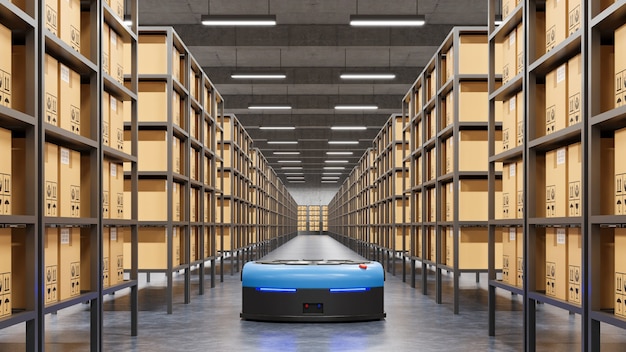The photograph depicts the interior of a meticulously organized, modern warehouse. Rows of metal shelving units, stocked with uniform yellowish-brown cardboard boxes, stretch endlessly into the background on both the left and right sides of the image. Each box features a consistent print, reinforcing the orderly appearance. The shelves narrow in perspective as they recede, emphasizing the depth of the warehouse. Above, two rows of fluorescent ceiling lights illuminate the scene, their rectangular forms similarly diminishing into the distance.

Central to the image is a sleek, autonomous robot with a blue top and a dark gray bottom, resembling a larger, industrial Roomba. It features a red button on its side and glowing blue lights at the front, and a screen on its gray portion. The concrete floor is smooth and gray, providing a clean pathway for the robot to navigate the orderly aisles. The entire scene, devoid of human presence, suggests a photo-op setup, highlighting the pristine and efficient environment.